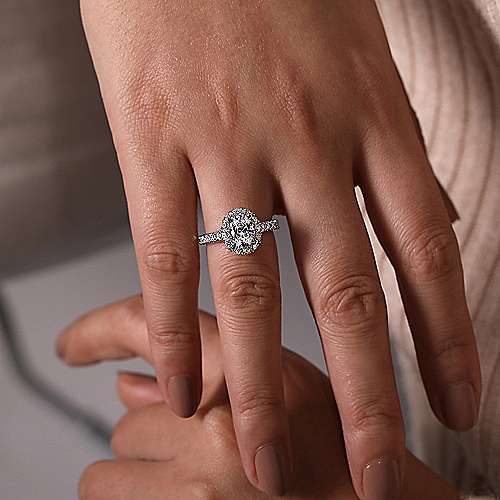The image showcases a close-up of a woman's right hand prominently displaying an engagement ring. Her hand, with neatly manicured nails painted in a light, neutral brown color, extends from the upper portion of the photo. The ring, worn on her right ring finger, features a large, sparkling oval diamond at its center, surrounded by smaller diamonds encrusted around the band. The metal appears to be white gold or silver. In the background, her left hand is visible but less prominent, with fingers partially hidden. The backdrop includes pink and brown striped cloth in the upper right corner, while the rest is a light brown or white. The focus of the image is the beautifully detailed, shiny engagement ring, meant to highlight its elegance and sophistication.